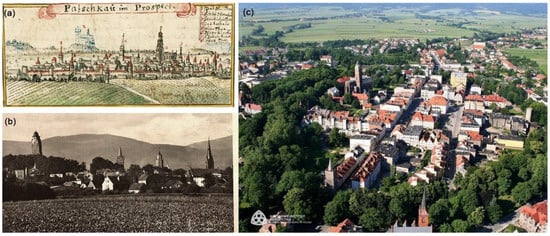This composite image features three different views of the same village, each labeled distinctly. 

In the top left, labeled 'A', there is an old, weathered sketch depicting an aerial view of the village. The drawing is detailed in pencil or possibly paint, outlining the basic structure of the village, including its white, tannish buildings with red roofs, and a surrounding expanse of farmland and roads. The atmosphere is historical, adding a picturesque charm with its grassy foreground and meticulously drawn buildings.

Below it, labeled 'B', is a black-and-white photograph capturing the village from a similar aerial perspective. This image shows more detail compared to the sketch, including some visible mountains and sky in the background. The familiar structures from image 'A' are also present, and the black-and-white format lends it an aged appearance, suggesting this photo was taken after the scene in 'A' but before the one in 'C'.

To the right, occupying a larger space under the label 'C', is a vibrant, live aerial photograph. This image presents the village in full color, revealing the true hues of the buildings with vivid red roofs and the lush greenery surrounding them. The scene includes numerous structures seen in both 'A' and 'B', along with expansive trees and fields encircling the village, indicating growth and development over time. The presence of tall monument structures further ties 'C' back to the previous images, providing a comprehensive evolution of the village landscape from sketch to modern-day photograph.